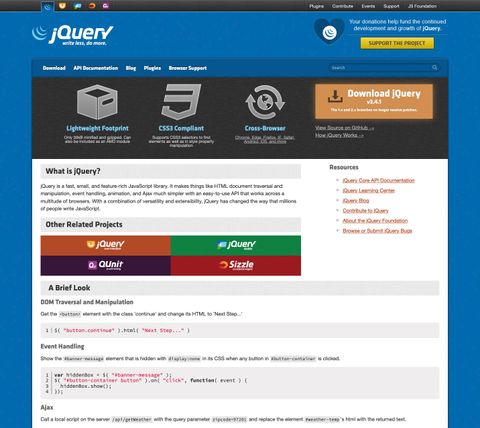The image depicts the homepage of the jQuery website, characterized by its tagline, "Write less, do more." On the right side of the page, there's a highlighted yellow button prompting users to "Support the Project" by making a donation towards the development and growth of jQuery. Accompanied by a heart icon enclosed in a circle, this call-to-action is prominently positioned. Below this section, a navigational menu offers links to various sections: Download, API, Documentation, Blog, and Support. Right beside these links is a search bar for additional accessibility.

Additionally, the lower part of the page features a segment with a black background, highlighting jQuery's advantages like "Lightweight footprint," "CSS1 Compliant," and "Cross-browser compatibility." In bold orange text, there's an option to "Download jQuery." Though the resolution of the website image is quite poor, which makes certain text difficult to read, it includes references to other associated projects, such as jQuery, QUnit, and Sizzle.